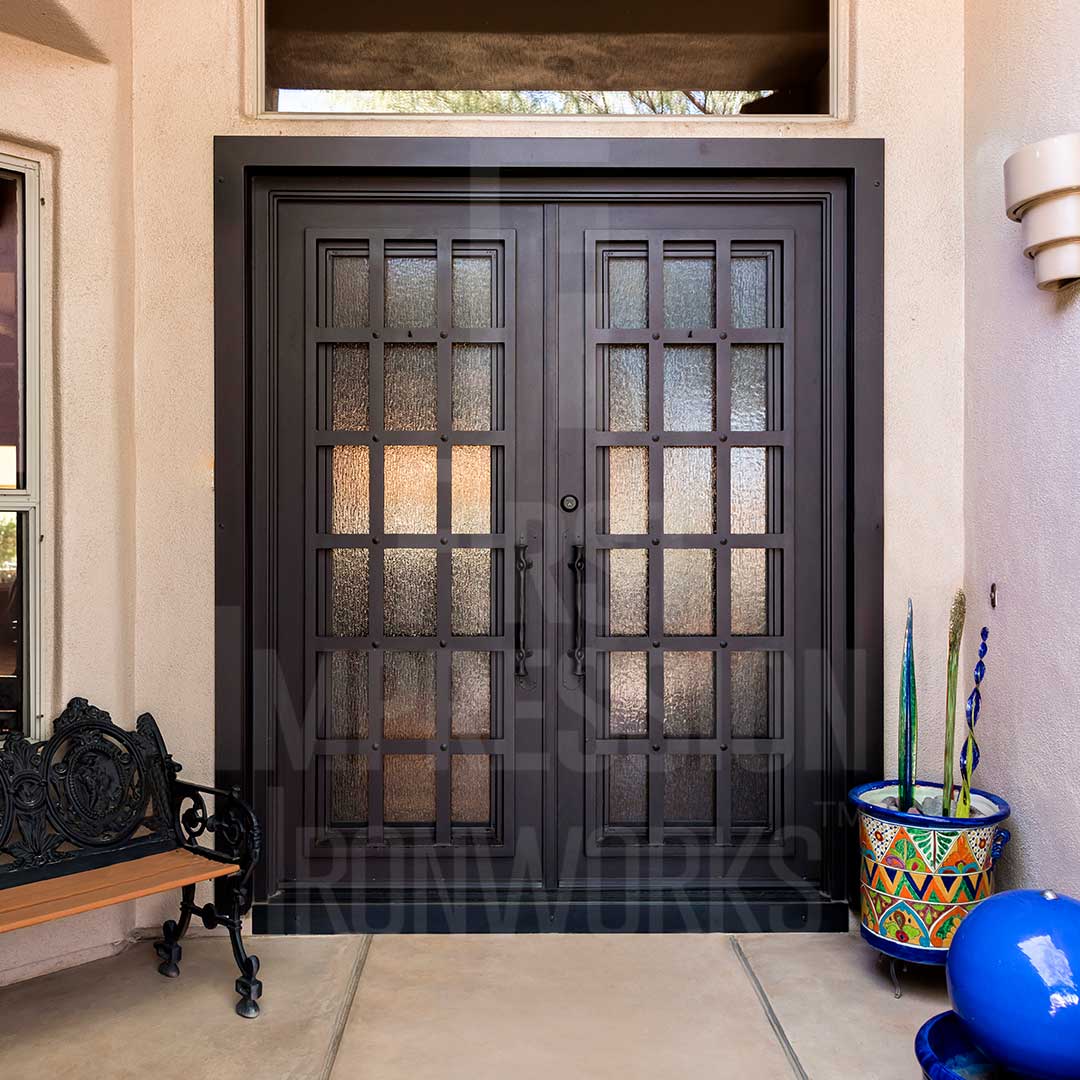This image depicts the front entryway of an elegant home, featuring double doors with distinctive design elements. Each door is a dark gray, adorned with multiple small glass panes framed in wood, creating a grid-like appearance. The handles on the doors are even darker gray, and one door includes a lock consistent with a deadbolt. Above the doors spans a large horizontal window.

To the left of the entryway, there is a bench resembling a park bench, constructed of wrought iron with a wooden seat. Adjacent to it stands a mosaic-type flower pot embellished with vibrant designs in blue, orange, white, and green triangular tile segments. Inside the pot are three stick-like decorations. Nearby, partially visible, is a bright blue, shiny, egg-shaped ornament resting in a matching blue base.

The floor is tiled in a peachy hue while the surrounding walls are a creamy white. A partially visible sconce light fixture with three circular layers is mounted on the right wall. Over the doorway, there is a watermark that reads, "Impression Ironworks," adding to the impression of a high-end residential entrance.